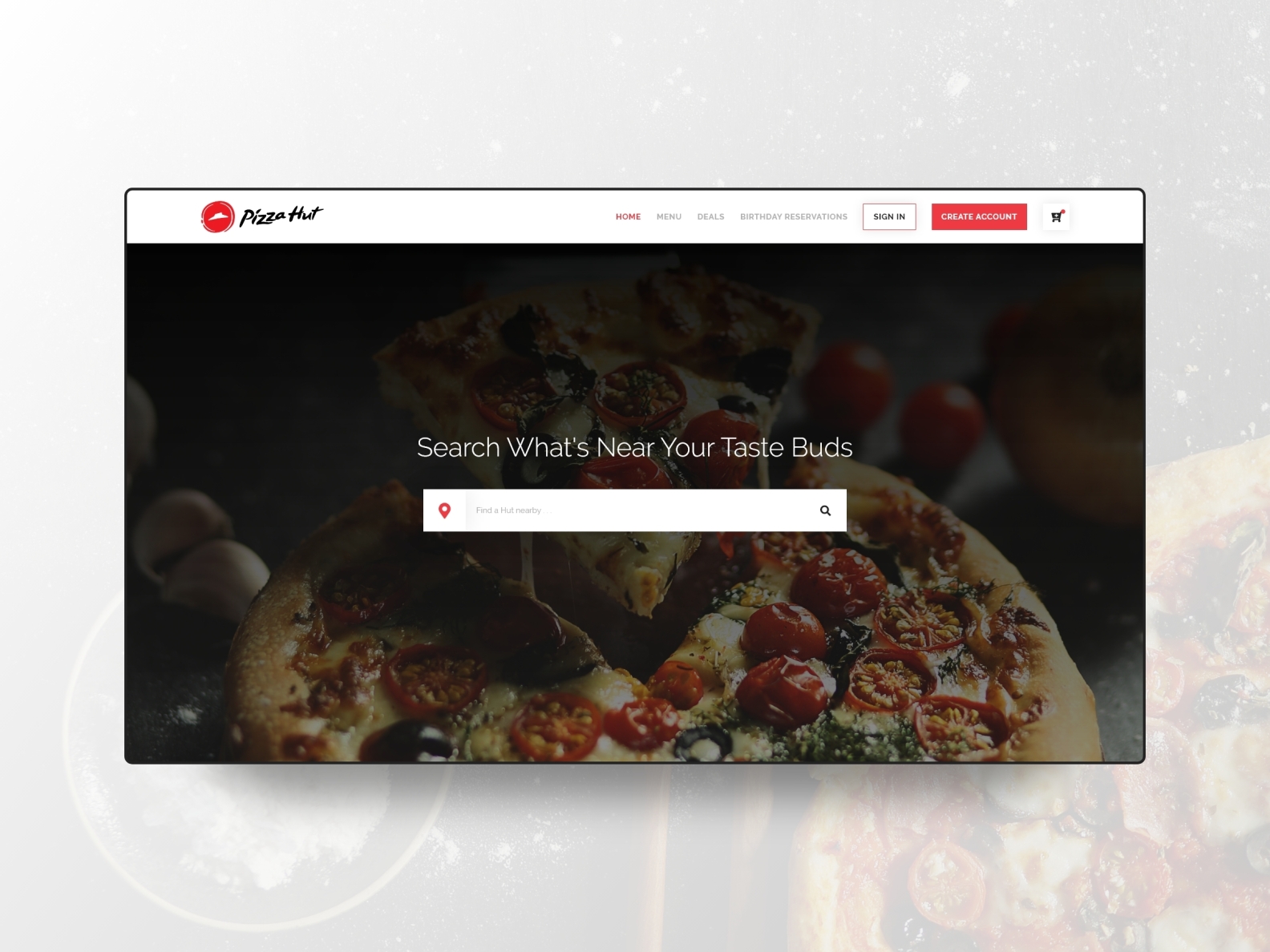The image depicts a sophisticated Pizza Hut interface against a light gray background with a pizza partially visible in the shadowed corner. The pizza in the bottom right corner shows a crispy crust, vibrant red sauce, dark green spinach, and slices of tomatoes, albeit subdued by the gray overlay.

Dominating the center of the image is a large, roughly square section, measuring about seven to eight inches on each side. At the top of this section, the iconic Pizza Hut logo is displayed: "Pizza Hut" written in bold black letters alongside a red circle containing a white hat symbol.

Adjacent to the logo, a menu bar features the following options in a sequence: "Home" highlighted in red, followed by "Deals" and "Birthday Reservations." To the right, a boxed text says "Sign In," paired with a contrasting red box labeled "Create Account." An icon of a shopping cart, encircled with a small red dot next to it, signifies the cart's status.

The focal point of the image is a well-defined pizza prominently placed at the center. The background surrounding the pizza is dark, making the toppings of cheese, tomatoes, and spinach pop visually. Above the pizza, the phrase "Search What's Near Your Tastebuds" invites interaction. Below this invitation lies a long search bar with a red circle to the right and an iconic magnifying glass symbol to the left, indicating its function.